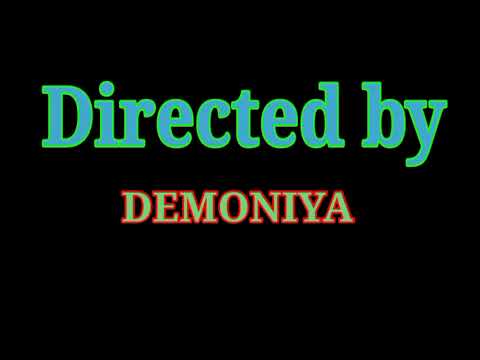The image is a landscape-oriented title block, typically appearing at the beginning or end of a film or video. It features a completely black background with centrally aligned, illustrated typography that is slightly closer to the top than the bottom. The first line of text reads "Directed by" in a large serif font, with an aqua blue color and a lime green outline. The "D" in "Directed" is capitalized, while the remaining letters are lowercase. The second line of text, "DEMONIAYA," is in all capital letters, with a light green color and a red outline. This title block serves as a stylistic credit slide, likely part of broader artwork that acknowledges various contributors to the film or video.